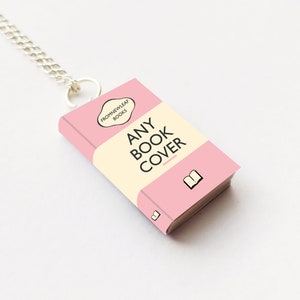The photograph showcases a charming book-shaped pendant, designed to look like a miniature book, placed on a white surface. The front cover of the pink pendant displays the title "any book cover" written across a cream-colored bar that stretches horizontally across the middle. Below this bar, there's a small open book icon adding to the bookish theme. This pendant is attached to a delicate silver chain via a silver ring, making it a dainty and literary piece of jewelry. The soothing pink hue of the charm, contrasted by the light beige central bar, creates an eye-catching and elegant necklace, likely favored by book lovers.